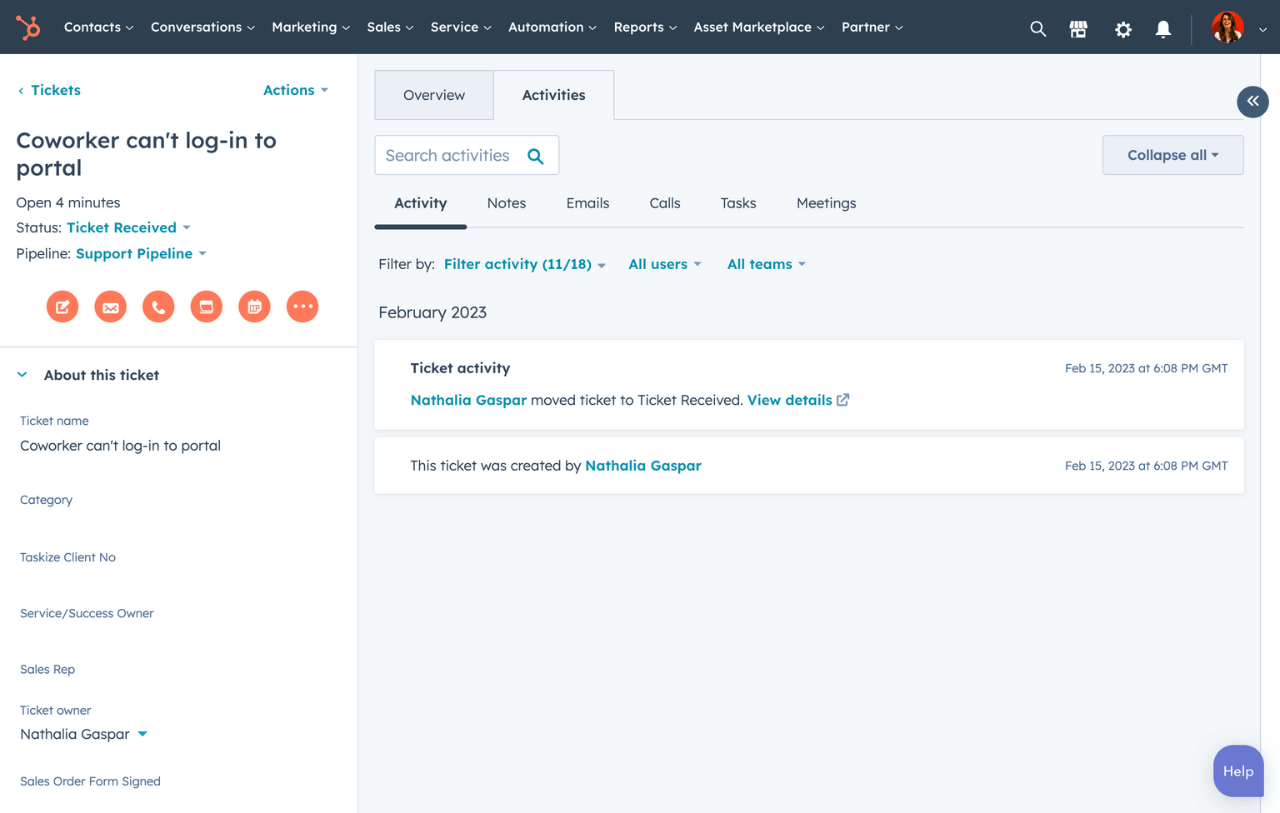This is a detailed and cleaned-up caption for the described image of the website interface:

---

The website interface features a comprehensive top banner, with several menu options for easy navigation. The top row includes:

- "Contacts" with a drop-down menu
- "Conversations" with a drop-down menu
- "Marketing" with a drop-down menu
- "Sales" with a drop-down menu
- "Services" with a drop-down menu
- "Automation" with a drop-down menu
- "Reports" with a drop-down menu
- "Asset Marketplace" with a drop-down menu
- "Partner" with a drop-down menu

To the right of the menu options, icons are displayed for additional functionalities, including a magnifying glass (search), a store or home icon, a settings icon, an alarm bell icon, and a profile picture with another drop-down menu.

Below the banner, the interface presents ticket management details. The first visible ticket shows:

- Ticket name: "Co-worker can't log in to portal"
- Status: "Open 4 minutes"
- State: "Ticket received"
- Pipeline: "Support pipeline"

There are six actionable icons next to the ticket for different interactions, including message, email, phone call, and three unspecified options along with an overflow menu.

The ticket details segment provides more information such as:

- Ticket name: "Co-worker can't log in to portal"
- Category
- Tasks list
- Client number
- Service/Success owner
- Sales representative
- Ticket owner: "Natalia Gaspar"
- Sales order status

In the main content section, the "Overview" and "Activities" tabs are present, with "Activities" currently highlighted. The activities tab allows searching through activities and comes with a "Collapse All" toggle. 

It shows six categories of recordable actions:

- Activities
- Notes
- Emails
- Calls
- Tasks
- Meetings

Filtering options include "Filter by" with a date range (11/18), all users, and all teams. The specific activity shown includes:

- Date: February 2023
- Activity: "Ticket Activity - Natalia Gaspar moved the ticket to 'Ticket received'"
- Option to view details of the activity
- Note that the ticket was created by Natalia Gaspar

Finally, a help button is located at the bottom right corner for user assistance.